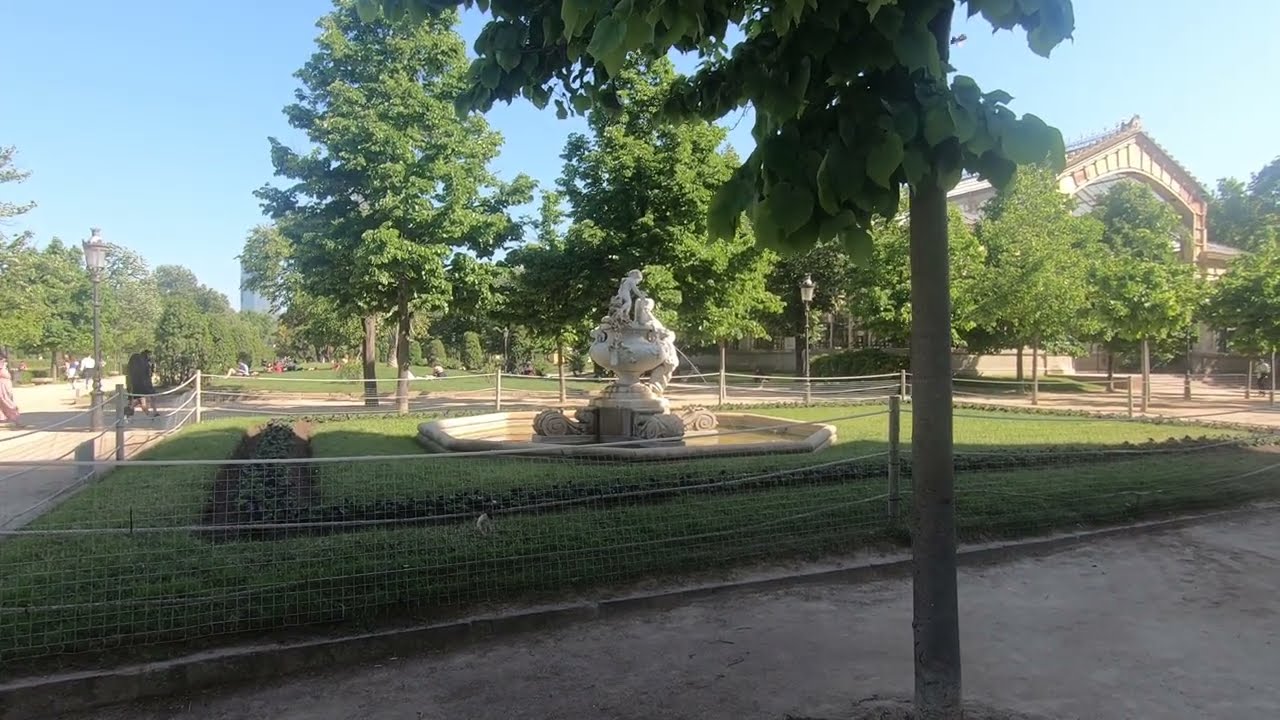This photograph, taken outdoors during the daytime, captures a small rectangular garden surrounded by a netted fence. The grass-covered garden features a cream-colored water fountain at its center, which appears to be hexagonal and adorned with a large bowl and playful children statues. At the lower left, a gray concrete pathway angles upwards, intersecting with a slender tree whose green, spade-shaped leaves extend down from the top of the image. To the right of the garden, additional trees and pathways are visible, along with street lights scattered throughout the surrounding area. The scene is bathed in sunlight, beneath a clear blue sky, and part of an arched building with a slanted roof can be seen in the background on the right-hand side. The combination of these details paints a serene, well-maintained outdoor space with a harmonious blend of natural and man-made elements.